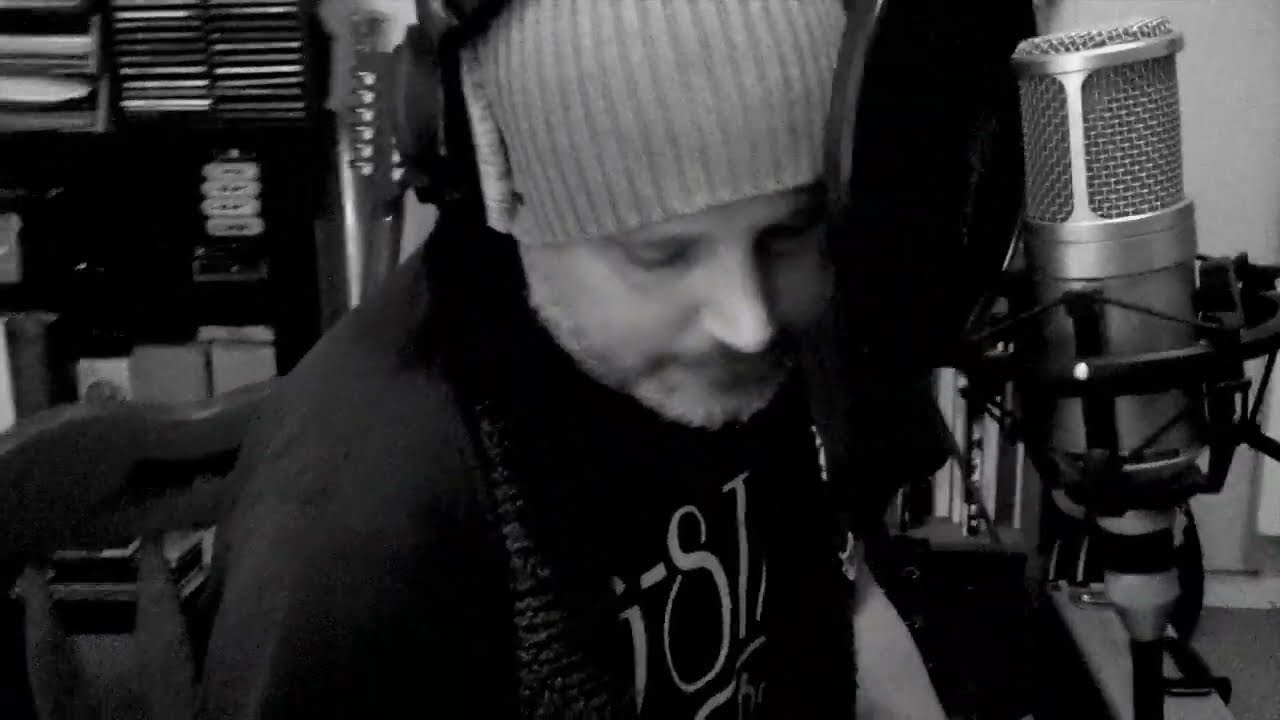This black-and-white photograph captures a man sitting in what appears to be a self-made recording area. The man, who is wearing a grayish beanie and dark clothes, has a slightly scruffy appearance with a beard and mustache that features some gray. He is equipped with headphones and is seated on a wooden chair. His head is slightly bowed, resting close to a microphone, which is positioned high on a mic stand and outfitted with a mesh wind guard. Behind him, there is a bookshelf filled with CDs and other miscellaneous items. The neck of a guitar is also visible, protruding from the left side of the frame. The detailed background and the casual seating arrangement contribute to the vibe of an improvised recording space rather than a professional studio.